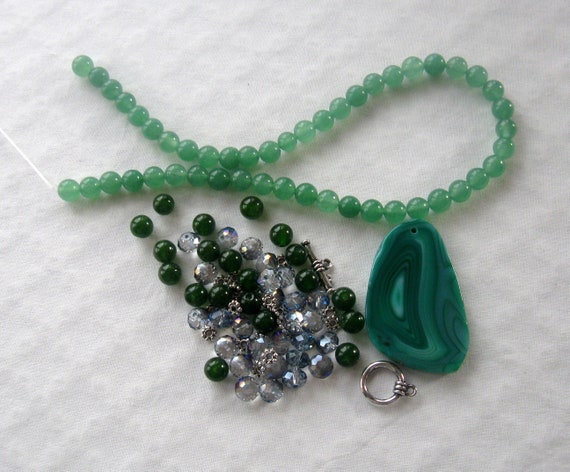The photo captures a collection of beaded jewelry meticulously arranged on a white cloth backdrop, which features faintly visible lines forming a subtle grid pattern. Central to the image is a necklace composed of light green beads that resemble jade or turquoise, forming a loose loop at the top and spreading out towards the bottom left, creating a shape reminiscent of a rudimentary fish. Surrounding the green beads are an assortment of additional beads, including black, clear, and gray variations, adding a rich texture and depth to the composition. Adjacent to the beads lies a prominent, polished piece of green material that echoes the jade-like aesthetic of the necklace. Beside it, a tiny, intricate ring with three smaller rings sits, contributing to the complexity and beauty of the display. The arrangement, possibly showcasing incomplete jewelry designs, highlights the craftsmanship and intricate details of the beaded creations.